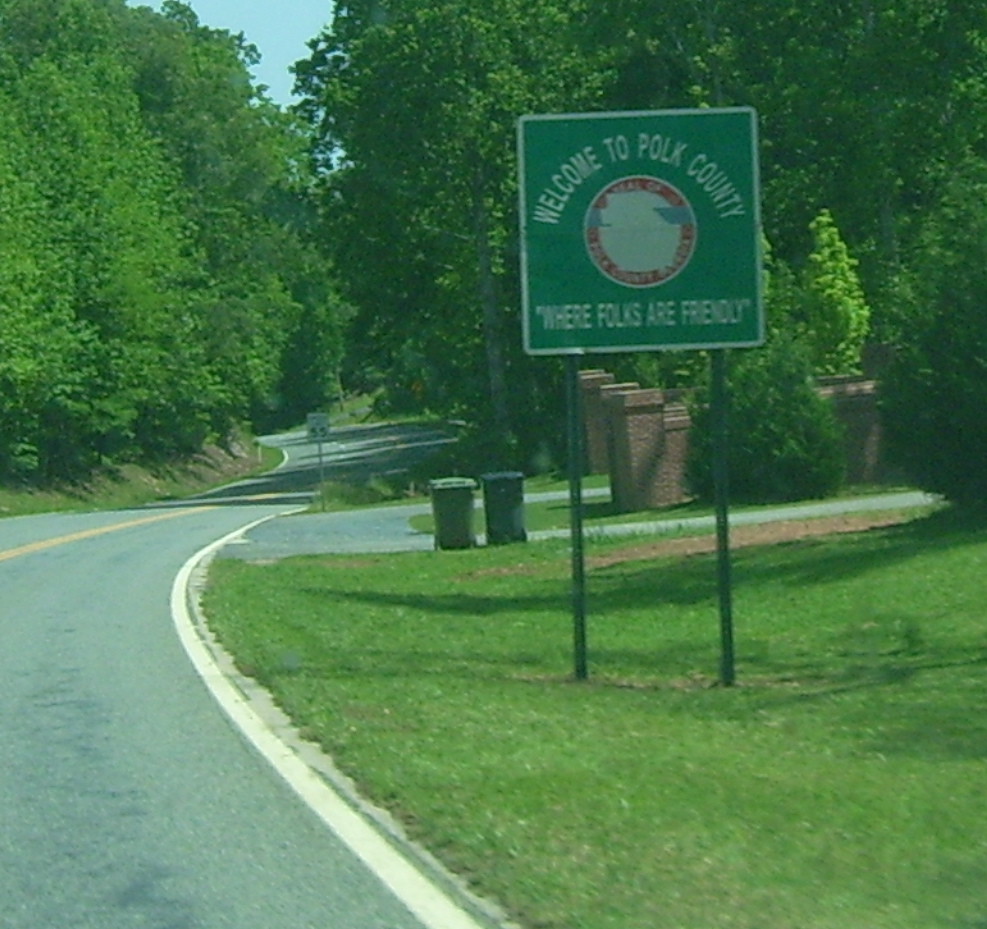This photograph captures a serene country road in a rural setting at the county line. Prominently displayed in the upper right portion is a green square sign with white lettering, welcoming travelers to Polk County. The sign features the County's seal or logo and a heartwarming motto that reads, "Where Folks Are Friendly," all supported by two narrow metal poles. Just behind the sign, an entryway and driveway to a home are noticeable, framed by a traditional red brick wall. Near the roadside, two garbage cans are positioned, emphasizing everyday rural life.

The road itself, positioned to the left of the image, runs with a single yellow line dividing the center and is noticeably absent of vehicles. In the distance, a 35 miles per hour speed limit sign can be seen, poised before the road gently curves to the left and disappears behind a thick screen of trees and lush foliage. The lower right quadrant of the image, in the foreground below the sign, shows a neatly trimmed grassy area, enhancing the overall picturesque and tranquil rural landscape.